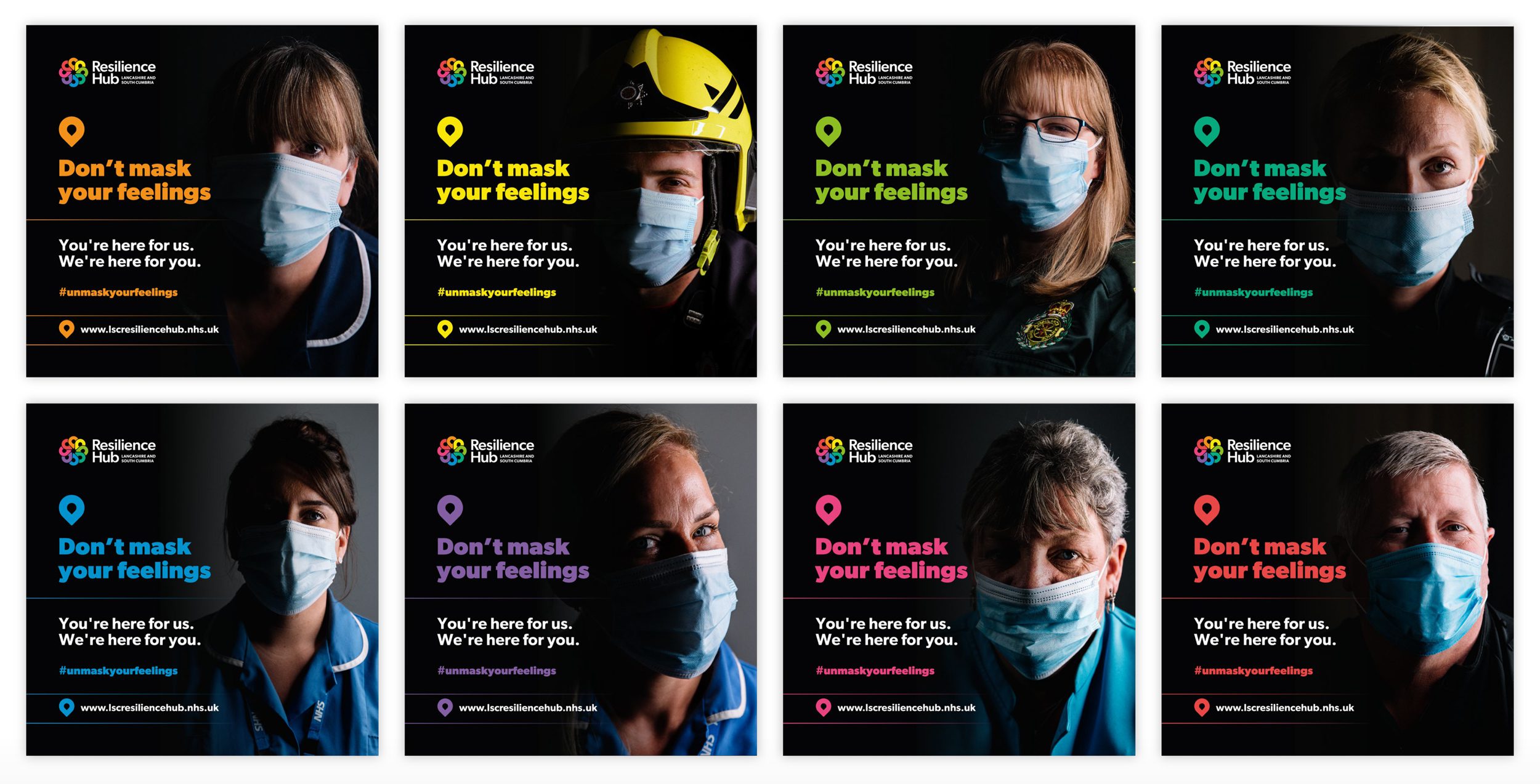This image features a grid of eight individual squares, each with a unique color background and the same uplifting message: "Don't mask your feelings." The squares are arranged in two horizontal rows. The top row includes squares in orange, yellow, lime, and teal, while the bottom row features blue, purple, pink, and reddish-orange colors. 

In all eight squares, on the right side, are people donning masks reminiscent of those worn during the COVID-19 pandemic. The individuals include five women and two men, with one man distinctively wearing a yellow helmet. Accompanying the message is a motivational text at the bottom: "We're here for you, you're here for us." 

The brand behind this poignant message is Resilience Hub, whose logo is represented by a circle filled with variously colored smaller circles, enhancing the theme of unity and support.